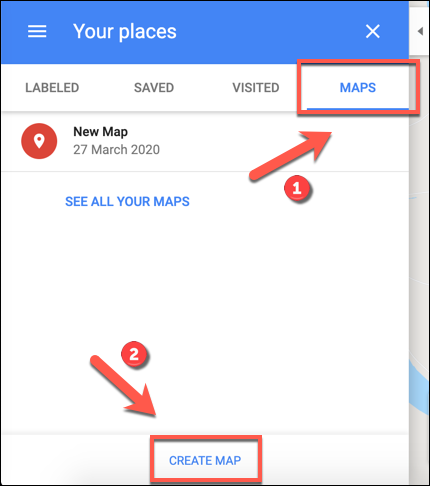This screenshot features a user interface with a predominantly white background and specific elements highlighted in blue and red for emphasis. At the top, a blue banner spans the width of the image. On the far left of this banner is an icon composed of three horizontal white lines, representing a menu. To its right, the text "Your places" is displayed in white. On the far right edge of the banner, there is a white 'X'.

Below the banner, the background transitions to white, and textual categories appear: "Labeled," "Saved," "Visited," and "Maps". The word "Maps" is colored in blue and enclosed by a red square. Adjacent to the word "Maps," a red circle contains a white pin icon indicating location. Below this icon, the text "New map, 27 March 2020" is visible.

A red arrow, labeled with the number "1", points upwards diagonally to the right towards the red-outlined "Maps" text. Beneath the arrow, the caption "See all your maps" is displayed.

Near the bottom of the screen, another red arrow labeled with the number "2" directs attention downward towards the center. Here, the text "Create map" appears in blue and is enclosed in a red rectangle, highlighting the button's functionality. This screenshot does not include any photographic content.